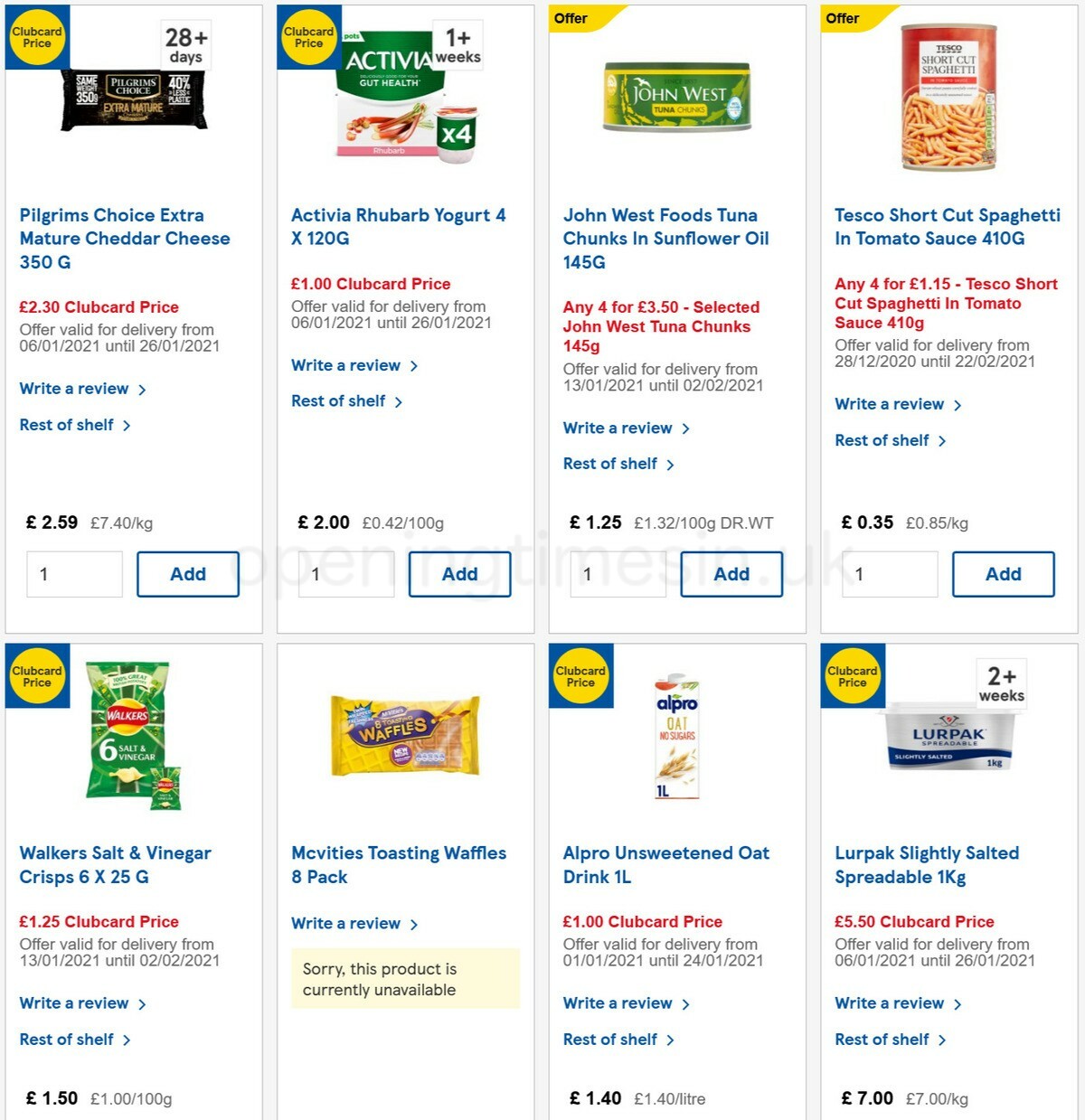Here is an enhanced and detailed caption based on the provided voice description:

In this image, we see a detailed snapshot of a digital food shopping interface, possibly displaying search results or a shopping cart. The interface is divided into four columns, each containing two product entries arranged vertically. 

Starting with the first item at the top-left, there is a product card for Pilgrim's Choice Extra Mature Cheddar Cheese. This card features a prominent 'Club Card Price Choice' icon—a yellow circle with a blue square around it. The product description includes detailed information such as the name, price, options for reviews, the ability to view the rest of the shelf, and an advertisement, along with a quantity selector.

Directly adjacent to this is another product under the same 'Club Card Price Choice' promotional banner: Activia Rhubarb Yogurt. Further to the right, we see a product card for John West Tuna, followed by one for Tesco Shortcut Spaghetti, completing the top row of items.

On the second row, the first product displayed is Walker's Salt and Vinegar Crisps, which also has the 'Club Card Price Choice' icon. This card includes a detailed section with reviews, shelf options, price, and quantity selector. 

Next, we have McBitie's Toasting Waffles 8-pack. Notably, this product is marked as unavailable and, therefore, lacks the usual review, shelf, or price details.

Wrapping up the bottom row of the interface are two additional products: Alpro Unsweetened Oat Drink and Lurpak Slightly Salted Spreadable. Each product card maintains a consistent layout, providing essential information such as the product description, price, and purchasing options, clearly aimed at creating a straightforward and informative shopping experience.